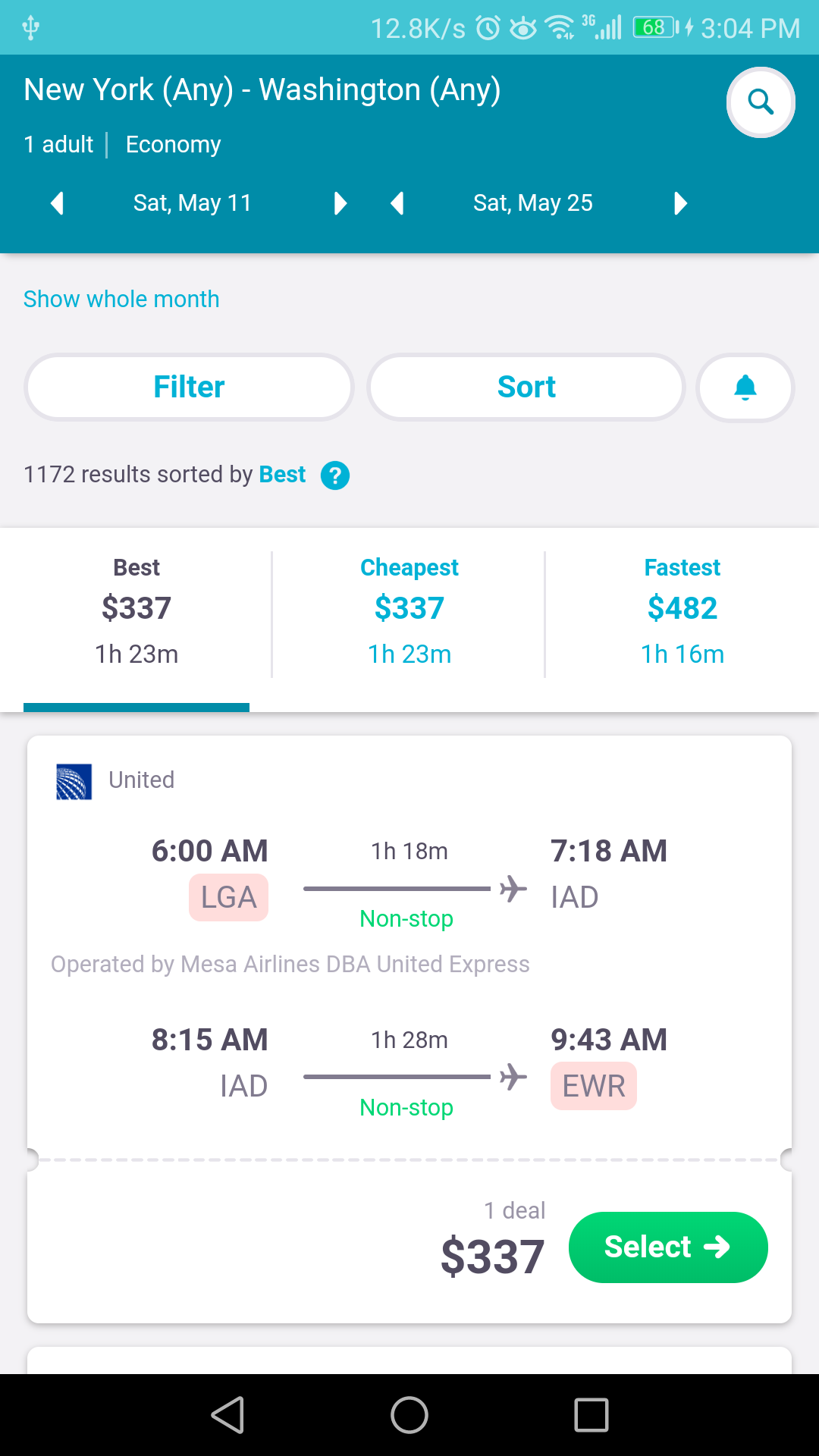This image displays a phone screen with an application open. At the top of the screen, various system icons are visible, including those for Wi-Fi, signal strength, battery level, and an alarm clock symbol. The time on the phone is displayed as "3:00 AM" and "4:00 PM," indicating the crucial times of interest or operations within the app.

The app interface prominently features information about a flight route, specifically detailing a journey from New York (NY) to Washington D.C. (DC). Below this information, the screen shows the travel dates, indicating a period from Saturday, May 11, to Saturday, May 25.

Additionally, the application includes functionalities for filtering and sorting search results, and currently displays a total of 1,172 results related to the user’s query or criteria. The interface appears user-friendly, displaying important details concisely for easy access and decision-making about the flight options.